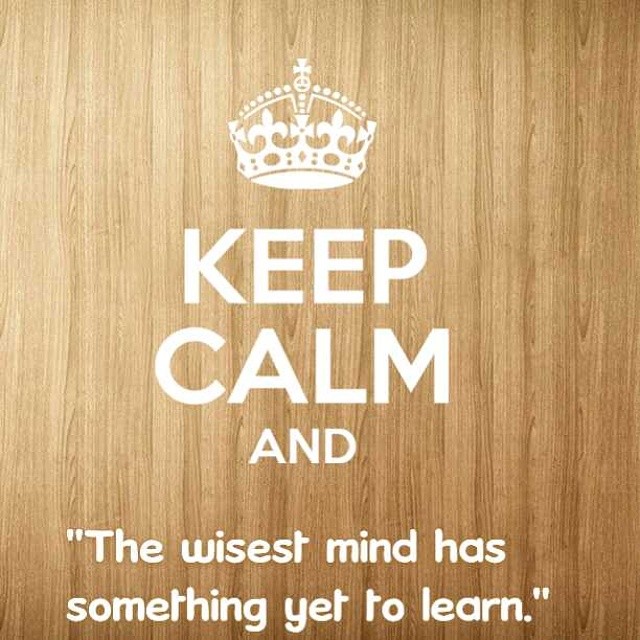The image features a light tan wooden background with vertical wood grain. Superimposed on the wood is a series of white, computer-generated texts and images. At the top, an ornate crown outlined in white is depicted, complete with a small cross and fleur-de-lis embellishments. Directly below the crown, in large, capitalized block letters, is the phrase "KEEP CALM." Following this, in a smaller, modern-style font with both upper and lower case letters, is the quote: "The wisest mind has something yet to learn." This text is spread across two lines and is placed near the bottom edge of the image. The overall design extends from corner to corner on the wooden surface.